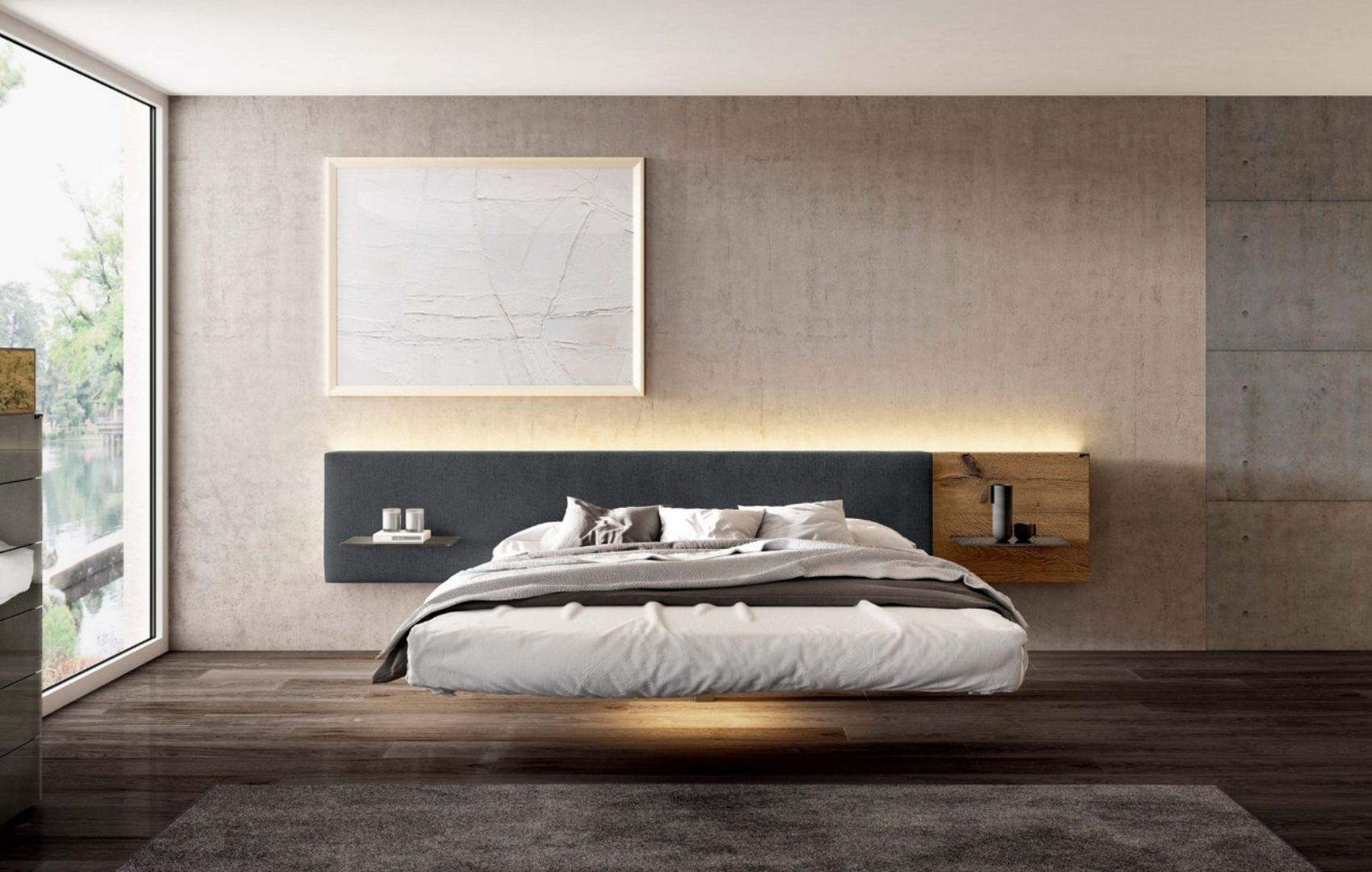This daytime photograph captures a meticulously arranged bedroom within a house. At the center is a bed appearing to float just above a wooden floor, covered with pristine white sheets, a gray blanket, and an additional darker blanket. Adorning the bed are three pillows: two white ones to the right and a darker one to the left. The gray headboard behind the bed transitions into a wooden segment on the right side, which may include speakers or other items. 

To the left, a large window allows natural light to flood the room, casting a warm glow on the beige-toned stone wall that shifts into gray wood paneling. A white-framed artwork graces the top left portion of this wall. A glass shelf, serving as a nightstand, holds a mug or thermos with a cup next to it. Additionally, a gray rug lays in front of the bed, adding to the room's tranquil ambiance. A dresser is visible toward the left, complementing the cohesive and cozy aesthetic of the bedroom.